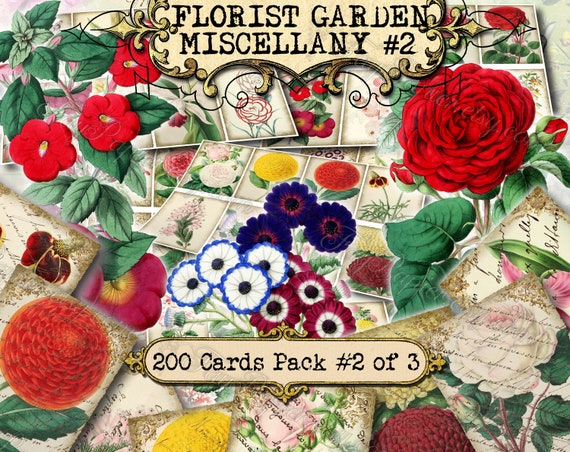The image depicts the top of a rectangular box with an ivory-colored background, featuring elegant black lettering that reads "Florist Garden, Miscellany Number Two." Prominently, it showcases an array of various flower illustrations, including red roses, blue flowers, white flowers, yellow flowers, and a distinctive red chrysanthemum in the top right corner with accompanying green leaves. Among the detailed floral designs, there are dark purple flowers with concentric circles of red and black in the center, and a white flower edged in blue, also with a black center. In black text below the illustrations, the box announces "200 cards, pack number two of three," emphasizing the variety and assortment of flower designs available in this set.